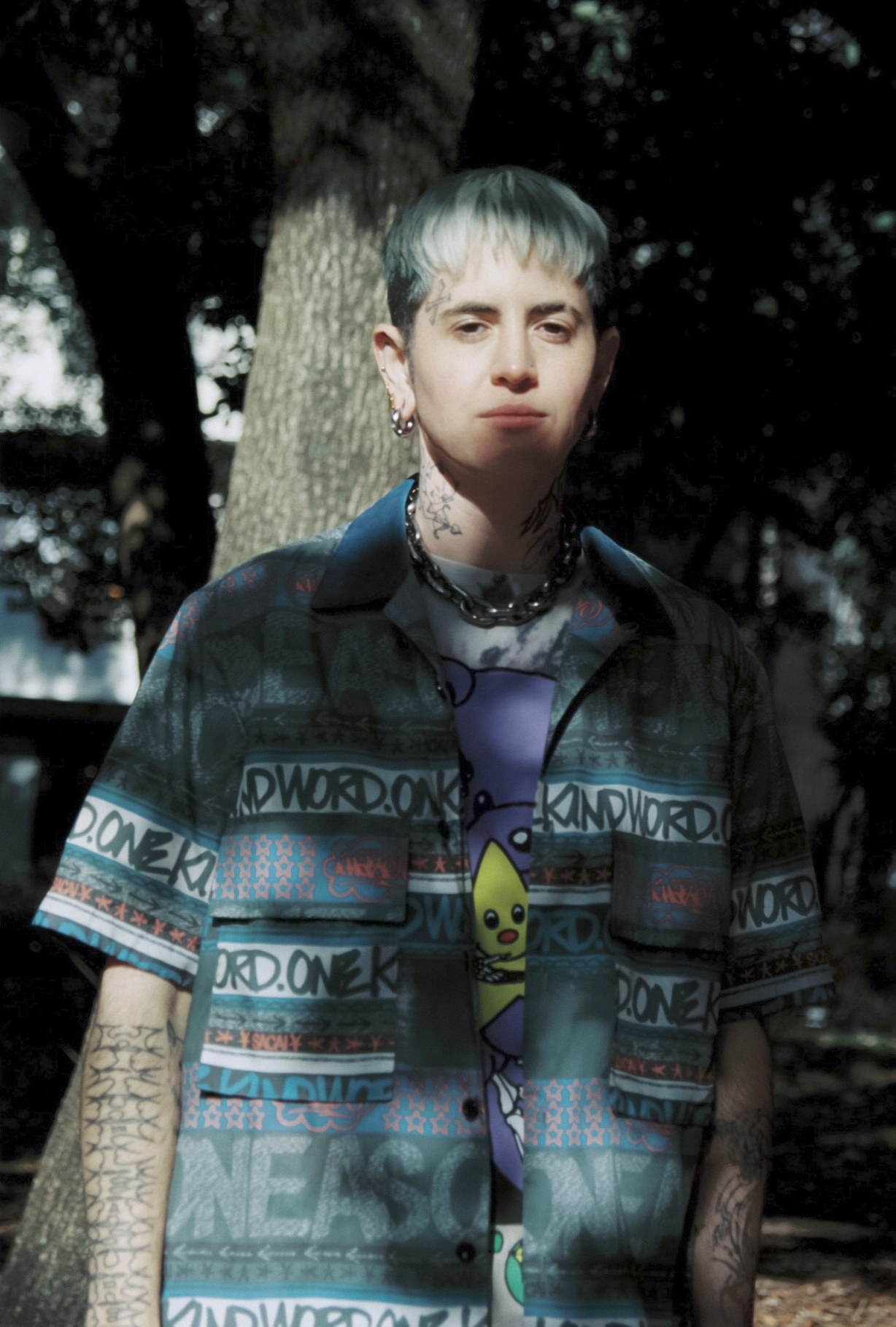In an outdoor setting, a striking photograph captures a young woman with a distinctive punk rocker style. She stands partially obscured by shadows created by sunlight filtering through the leaves of a large tree behind her. Her short, fashionably styled hair contrasts sharply in color, being bleached white at the front and jet black along the shaved sides. Despite the dim and somewhat desaturated tone of the image, her unique features stand out vividly.

The woman gazes directly at the camera with a serious expression, her face adorned by a small tattoo resembling an 'X' above her right eyebrow and a noticeable slit in her eyebrow. Numerous earrings decorate her ears, and tattoos subtly mark both sides of her neck and run along her forearms, featuring curved, intricate designs.

Her attire is equally eye-catching: she wears a heavy silver chain necklace and a layered ensemble comprising a short-sleeved blue button-down shirt over a purple t-shirt. The t-shirt showcases a yellow cartoon character with a tapered dome head amidst a backdrop of various words and letters arranged in bands across the fabric. The letters spell out seemingly random sequences such as "D-O-N-E-K-I-O-R-D," "D-W-O-R-D-O-N-K-I-K-N-D," and "V-O-R-D-N-E-A-S-C-O-D-O-N-N-O-N." The visual composition is punctuated by the tree and a gray sky that form the blurred background, enhancing the overall atmospheric quality of the photograph.